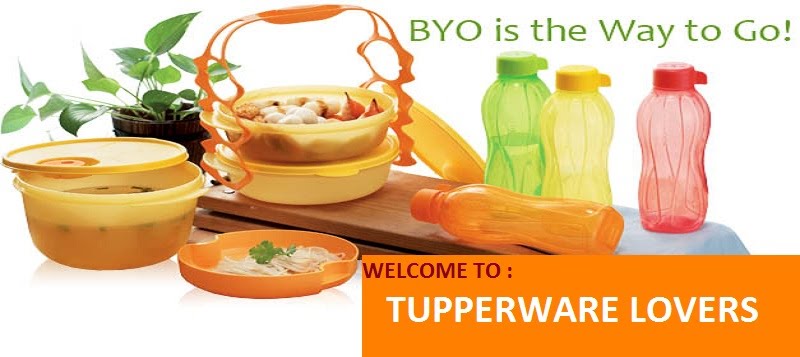The image prominently features an assortment of colorful Tupperware containers and bottles, arranged on a surface that looks like stacked pieces of wood, possibly in a kitchen setting. The title text at the top of the image, “BYO is the way to go,” is displayed in vibrant green, emphasizing the encouragement to bring your own containers. Below it, there's a green potted plant with broad leaves positioned to the left. Beside the plant, there's a set of two round plastic containers with orange handles, stacked vertically. The top container is open, revealing nuts and figs, while the bottom container is closed. In front of the plant, part of a bowl of soup in a slightly open plastic container is visible. To the right, there are four plastic bottles in various colors: orange, green, yellow, and pinkish-red, one of which is lying down. An additional piece of text on an orange rectangle at the bottom right reads, “Welcome to Tupperware lovers,” with the phrase “Welcome to” in purple or burgundy and “Tupperware lovers” in white. The entire scene is set against a wooden background, evoking a cozy and organized kitchen atmosphere.